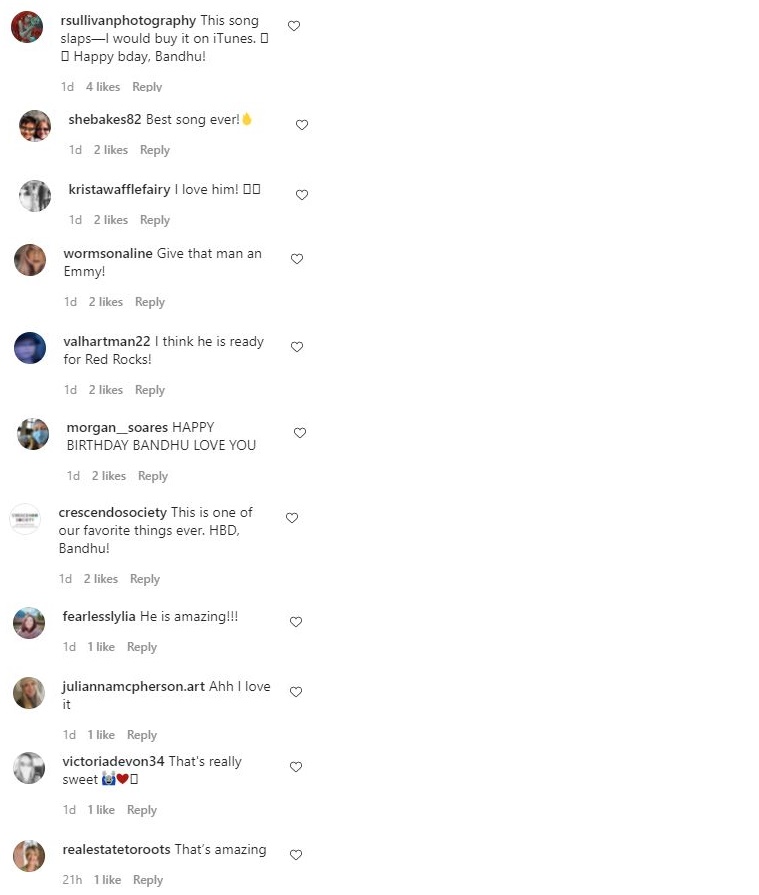A screenshot captures a white background featuring a series of text messages, each enclosed in a rectangular box. The messages express admiration and enthusiasm for a song with comments such as, "This song slaps, I will buy it on iTunes," "Best Song Ever," and "I think he is ready for Red Rocks." Additionally, there are birthday wishes addressed to someone named Bendu with messages like "Happy B-Day, Bendu," "Happy Birthday Bendu, Love You," and "HBD, Bendu." Repeatedly, the phrase "I love him" appears alongside supportive comments like "Give that man an Emmy" and "This is one of our favorite things ever." Each message is accompanied by user engagement metrics, indicating likes and replies.